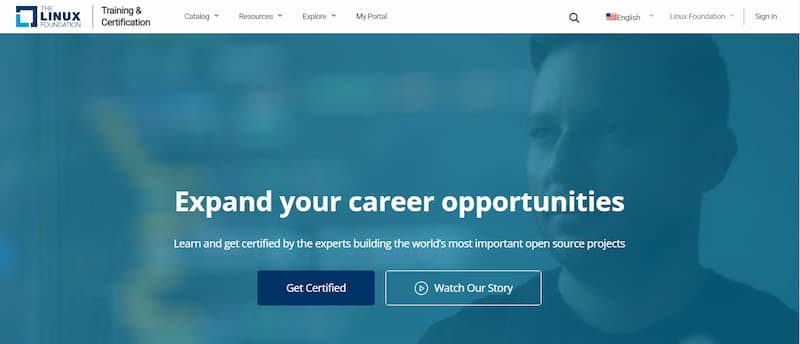**Detailed Caption:**

The webpage belongs to the Linux Foundation, identifiable by its logo in the upper left corner. The logo consists of a dark blue square symbol and text with "Linux Foundation" in a mix of dark and light blue colors. The main navigation bar at the top of the page includes four tabs: Catalog, Resources, Explore, and My Portal. There's also a magnifying glass icon, presumably for the search function, and the website is set to English, indicated by a small English flag. The page prompts users to sign in.

In the central part of the page, a semi-transparent blue overlay reveals the image of a middle-aged white man, possibly in his 40s, with a beard. His face and a portion of his shirt are visible, though the blue overlay obscures finer details, suggesting he's behind a glass-like filter. The background is slightly blurred, hinting at an office setting.

The prominent headline reads, "Expand your career opportunities. Learn and get certified by the experts building the world's most important open source projects." Below this text are two primary action buttons: "Get Certified" in dark blue with white text, and "Watch Our Story" in white text with a white rectangular outline and a play button icon, likely indicating a video.

Overall, the page maintains a professional and clean design on a white background, reinforcing the Linux Foundation's focus on training and certification.